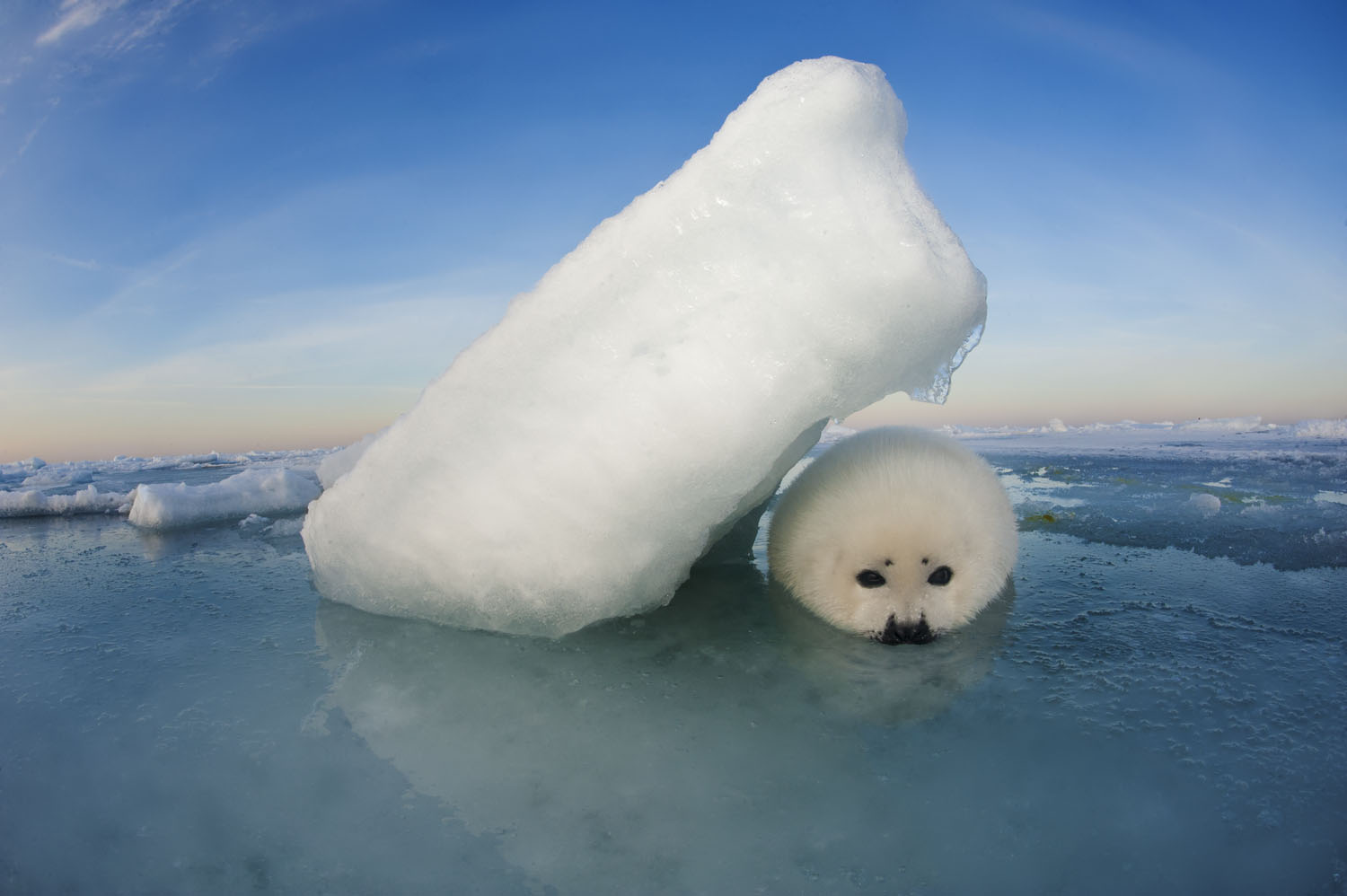In this captivating nature photograph, we find ourselves in an Arctic wilderness. The foreground features a patch of ice, interspersed with chunks of snow resting peacefully atop. Dominating the scene is a large, rectangular slab of ice that slopes diagonally from the bottom left to the top right. Beneath this icy overhang, a baby seal lies huddled, its entire white, fluffy form stretched out on the ice. The seal’s small black eyes and delicate black nose stand out against its white fur, giving it a serene expression as it faces the camera.

To the right of the seal, a small green patch of earth hints at the sparse vegetation in this frozen landscape. The background showcases a band of icy water, peppered with floating ice floes, under a clear blue sky adorned with a few wispy clouds. The horizon is accentuated by a subtle blend of orange and white hues, creating a breathtaking backdrop to this serene Arctic scene.